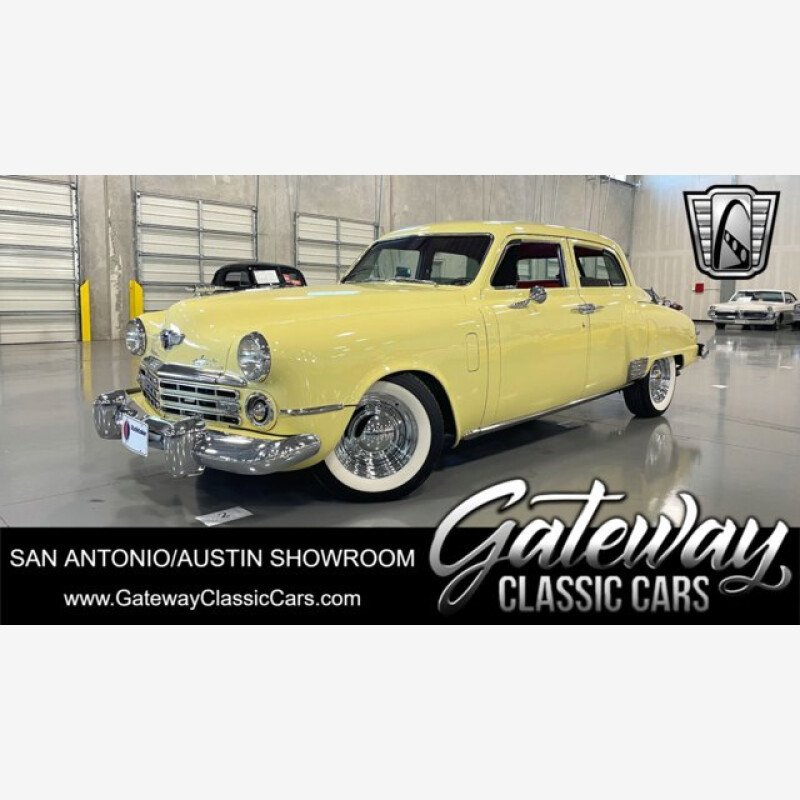The image showcases an elongated, classic yellow car from the 1950s, centrally positioned and slightly diagonal to the left within a large, garage-like showroom. The showroom features shiny, dark gray concrete floors that reflect the car and has gray walls with a row of white garage doors visible on the left-hand side. The car's exterior boasts numerous chrome details, including a large front bumper, a chrome grille, and rounded headlight casings. The vehicle features suicide doors, distinguished by their inward-opening handles. The wheels are notable for their chrome hubcaps and white wall tires. Adjacent side mirrors are also chrome-plated. At the bottom of the image, text reads: "San Antonio / Austin Showroom, Gateway Classic Cars, www.gatewayclassiccars.com," suggesting it is part of an advertisement for the showroom. The overall bright yellow hue of the car, combined with its reflective surroundings and detailed chrome finishes, highlight its vintage elegance and pristine condition.